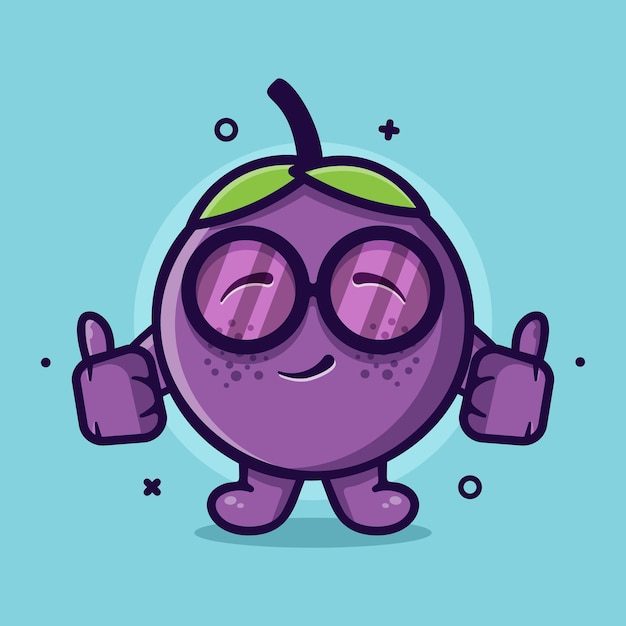The image is a humorous, cartoon-style drawing with a teal background. Central to the image is a round, purple character that resembles a grape or blueberry, outlined in black. The character has a cheerful demeanor, indicated by its half-smiling, comma-shaped mouth and squinting eyes. It sports large, round, dark purple glasses encircling its expressive eyes, along with light purple freckles scattered across its face. On top of its head sits a short purple stem, flanked by two green, leaf-like appendages resembling an alarm clock's bells.

The character's stubby arms extend to the sides, each hand giving a thumbs-up gesture. It stands on short legs with small feet. Surrounding the character, arranged in a circular pattern, are various black symbols: a dot (circle) and a plus sign directly opposite each other to the left and right respectively, another set of a dot and a plus sign (or X) opposite each other below, enhancing the playful and symmetrical composition of the image.